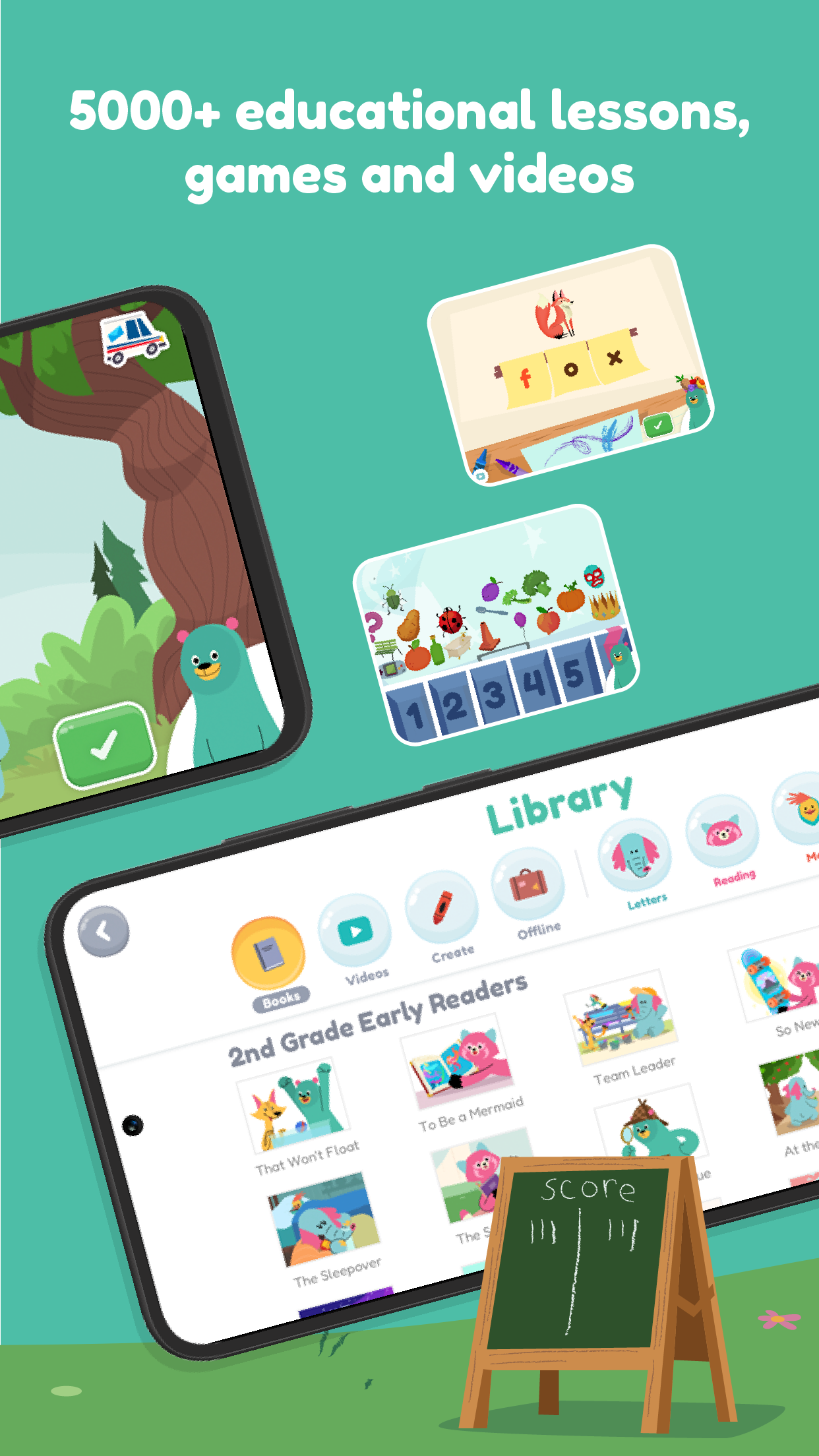The image displays a vibrant and engaging advertisement for a children's educational mobile application. The background color is a bright turquoise, evoking a playful and child-friendly atmosphere. At the top of the image, white text announces "5,000+ educational lessons, games, and videos," emphasizing the extensive resources available through the app.

Central to the advertisement are images of smartphones showcasing the application's interface. On one phone screen, the app's library section is visible, featuring categories like "Books," "Videos," "Create Offline," "Letters," "Reading," and a dedicated section for "Second Grade Early Readers." Example book titles listed include "Team Leader," "We Have to Be a Mermaid," and "The Sleepover."

Above the phone images, there's a depiction of an animated forest scene, complete with clickable buttons and a bear in the backdrop, likely representing one of the interactive learning environments within the app.

At the bottom of the advertisement, a small scoreboard is visible, marked with a '3' on both sides, though its specific function is unclear. The clean, colorful design of the advertisement, coupled with its focus on educational content, suggests a well-developed tool for parents seeking to support their children's learning and development.